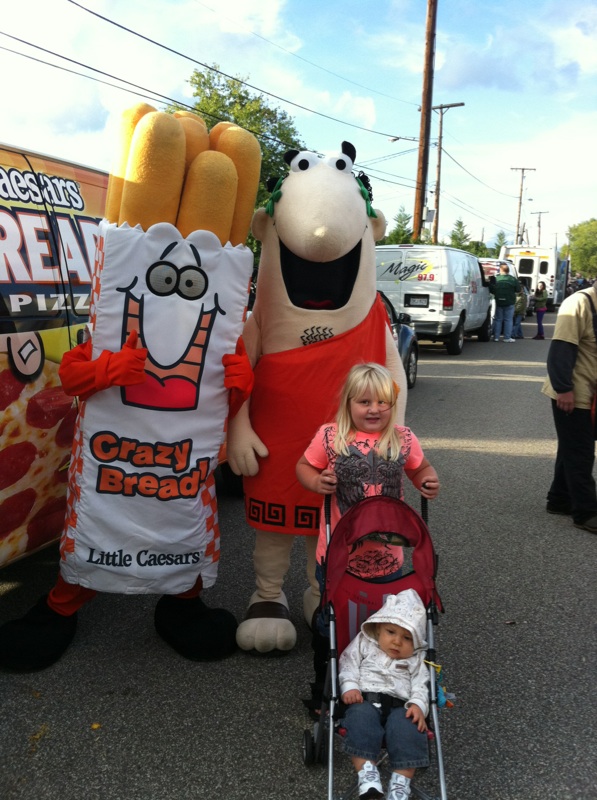The image is a color photograph in portrait orientation capturing a lively street scene during a food truck gathering, possibly a parade. The main focus is on the foreground, where a young blonde girl, around five years old, smiles as she pushes a red stroller with a young boy sitting inside. The boy is dressed in a white hooded sweatshirt, jeans, and white shoes. Standing behind them are two mascots from Little Caesars. The mascot on the left resembles a white bag with a face and breadsticks sticking out of the top, and it has the words “Crazy Bread!” written in orange on the front. The other mascot, to the right, is dressed as Little Caesar in a toga. Both mascots are engaging with the children, with the Crazy Bread mascot giving two thumbs up. Behind the mascots is a Little Caesars van adorned with the company’s logo and branding. In the background, the horizon is dotted with several other food trucks and vans, including one from Magic 97.9, as well as people mingling around. Overhead, there are street poles, trees, a blue sky, and some clouds. The image evokes a sense of community and festivity with its detailed representation of the scene.